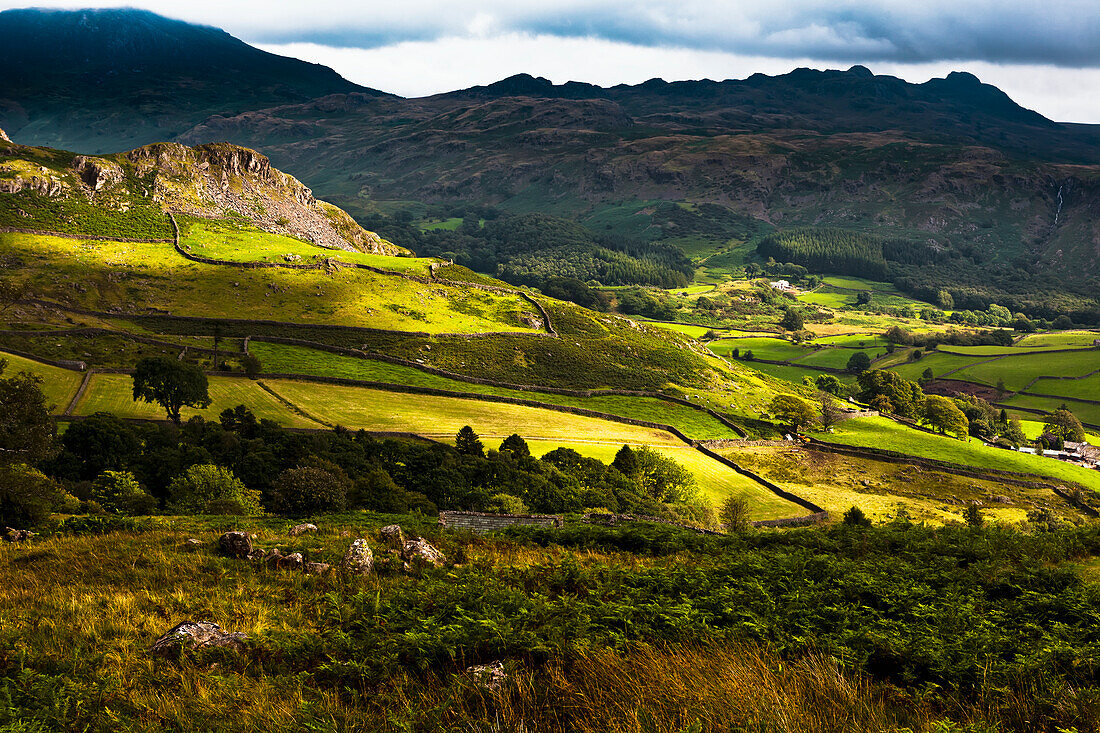This captivating landscape photograph captures the serene beauty of a secluded countryside. At the forefront, lush green fields stretch expansively, showcasing a picturesque patchwork of varying shades of green, from vibrant light hues to deep, rich tones. The fields are dotted with an abundance of robust, verdant trees, their foliage appearing particularly vivid and healthy, further enhancing the scene's natural allure. Stone walls, dark gray with hints of brown, intricately weave through the fields, subtly sectioning the landscape.

In the distance, the terrain transitions seamlessly into rolling hills and majestic mountains, their rugged forms painted in earthy browns and deep greens. The mountains provide a dramatic backdrop that accentuates the depth and tranquility of the scene.

Above, a sky blanketed in thick, bluish-gray clouds casts a soft, diffused light over the landscape, creating a serene and somewhat ethereal ambiance. The overall composition captures the timeless beauty of rural life and the undisturbed splendor of nature.